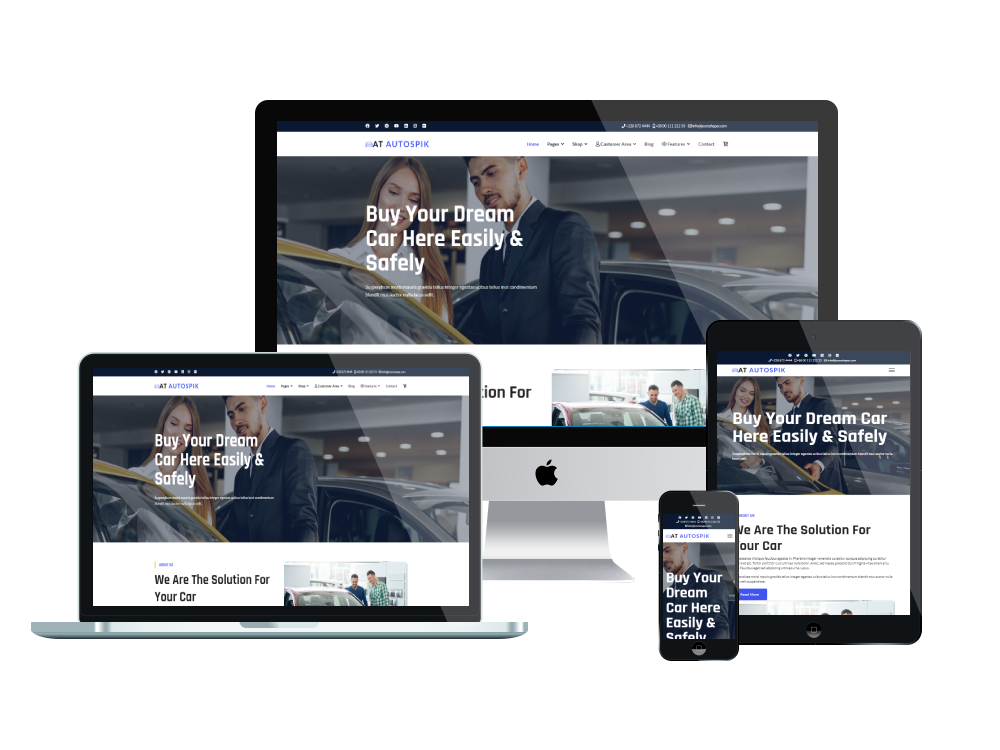In the image, there is an array of technology devices showcasing various views of an online car-buying website. A prominent Apple desktop monitor in the background displays the site with a headline, "Buy Your Dream Car Here Easily and Safely," featuring a picture of a woman, a man, and another woman inspecting a tan-ish yellow car, with a gray car parked behind them. Below the monitor, two men are examining another car. 

Adjacent to the desktop monitor, a laptop screen mirrors the exact same webpage, emphasizing the seamless cross-device experience of the website. Additionally, an iPad screen depicts a slightly different version of the page: the man and woman are positioned at the top, accompanied by a text overlay that says something akin to "the solution for your car" with a prominent purple bar on the left side. Finally, an iPhone screen shows a more condensed version of the site, focusing solely on the man looking at the car with the headline, "Buy Your Dream Car Here Easily". 

The collection of devices, set against the backdrop of a showroom illuminated with recessed lighting, illustrates how the website dynamically scales its content to fit various screen sizes, providing an adaptable user experience from the largest desktop view down to the smallest mobile display.